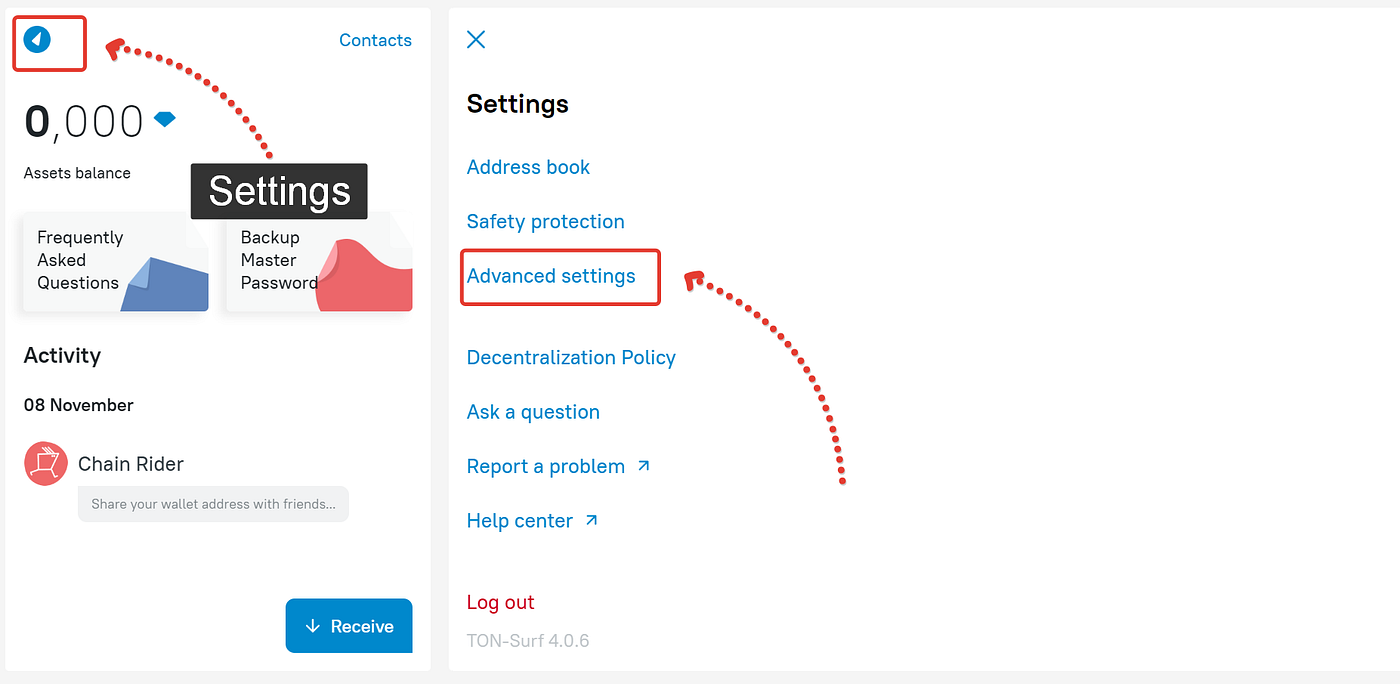Screenshot of a Cryptocurrency Wallet User Interface

The image reveals a neatly organized user interface of a cryptocurrency wallet application. The main dashboard, predominantly situated on the left side, features a clean and minimalistic design with a light blue and white color scheme. 

Prominently displayed at the top left is a blue logo icon. Below the logo, the dashboard lists the user's asset balance, currently showing 0.0000 tokens. Several buttons are positioned beneath the balance: one for frequently asked questions (FAQ) and another to back up the master password. 

The dashboard further includes an activity section, showcasing a single entry dated November 8, labeled "Chain Writer Receive." A blue "Receive" button is located at the bottom of this section.

On the right side of the image, the settings menu is expanded, displaying various options: Address Book, Safety Protection, Advanced Settings (highlighted and accentuated with a red text box and arrows, indicating it is either selected or of primary focus), Decentralized Policy, Ask a Question, Report a Problem, Help Center, and Log Out.

Overall, the user interface appears user-friendly, methodically arranged, and aesthetically pleasing with its consistent light blue and white color scheme.